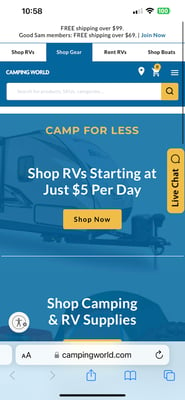Screenshot of Camping World Website for Camping Supplies

The screenshot captures the homepage of Camping World, a popular website for purchasing camping and RV supplies. The top status bar displays the current time as 10:58, indicating the user's active cellular service icon, Wi-Fi connection icon, and a green battery strength icon.

A prominent banner at the top of the webpage states, "Free Shipping Over $99," enticing potential customers. Below this banner, the website offers multiple navigation menus titled "Shop RVs," "Shop Gear," "Rent RVs," and "Shop Results." These are designed for easy browsing of various camping-related products and services.

In the center of the page, there is a search bar for users to find specific items quickly. The background transitions to a blue theme, featuring an image of an RV or camper with a headline "Camp for Less." The text accompanying the image advertises, "Shop RVs starting at just $5 per day," emphasizing affordability. Two prominently displayed yellow buttons are available for user interaction: a horizontal "Shop Now" button and a vertically aligned "Live Chat" button with a speech bubble icon, offering instant customer support.

Further down, another section reads "Shop Camping and RV Supplies," guiding users towards more specialized camping necessities.